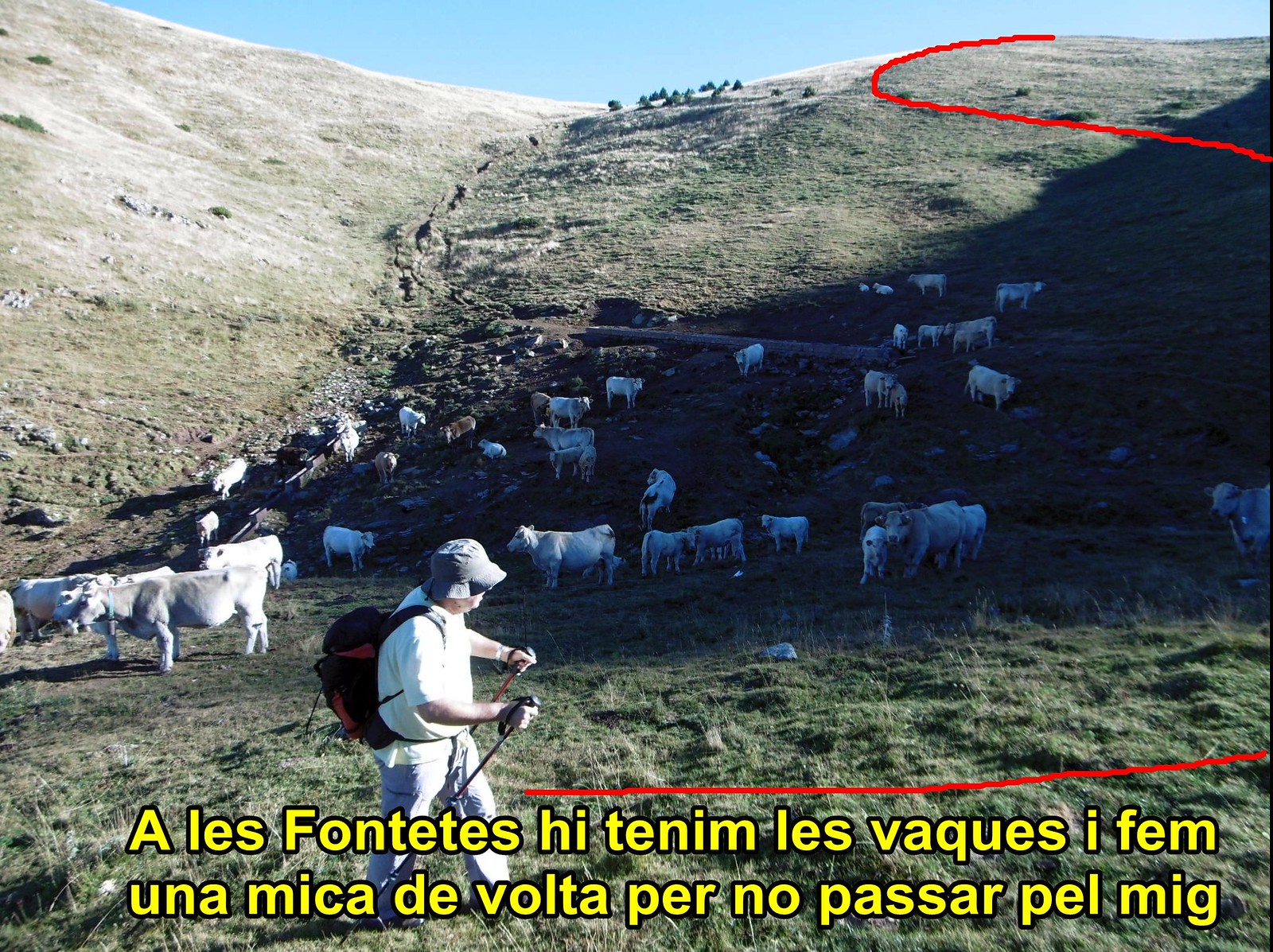The photograph captures a picturesque scene of a man hiking across a vast, grassy hill, accompanied by a herd of cows scattered around the landscape. The hill's grass appears vividly green on the right side, contrasting with the drier, less verdant grass on the left. The sky above is a clear blue, adding to the serene atmosphere. At the foreground and slightly to the left, the hiker—a man wearing a green or visor hat, a white polo shirt, and light brown or grey pants—is clearly visible. He sports a red and black backpack and is equipped with two hiking sticks, suggesting a prepared and purposeful trek. Despite the absence of snow, his equipment is reminiscent of skiing gear, possibly for navigating the damp or marshy terrain. The image features yellow text superimposed at the bottom, written in a different language, reading: "A les fontes y tenem les vaques a fem una mica de volta per no pasar pel mig." This text adds an additional layer of intrigue, complementing the natural and rustic charm of the scene.